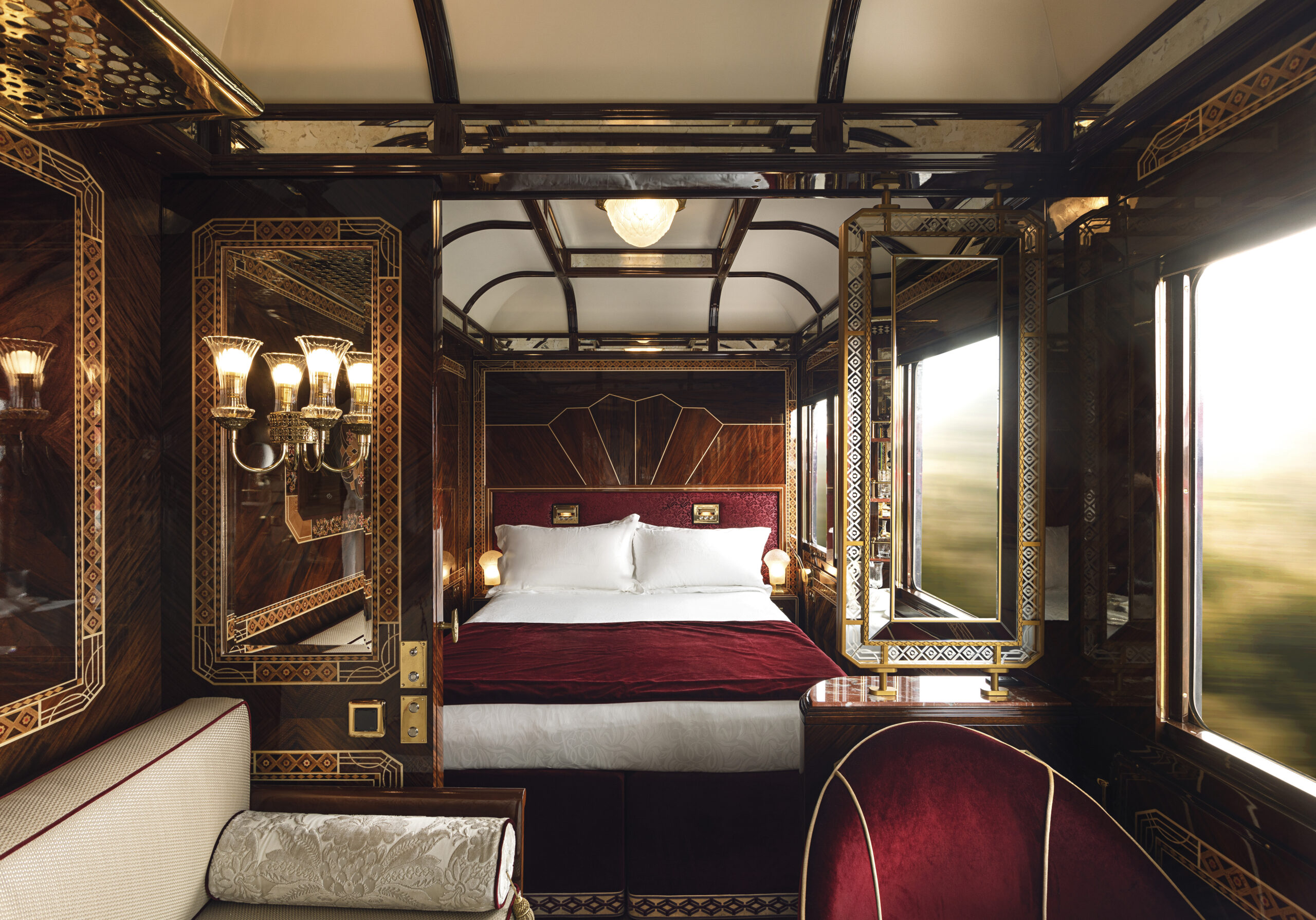The image captures an opulent bedroom situated in a luxurious train suite. Dominating the scene is a large bed adorned with pristine white sheets and two white pillows, complemented by a neatly folded red velvety blanket at its foot. The bed boasts an elaborate floor-to-ceiling headboard, intricately designed with wood, gold, and red elements. On the left side of the image, there's a beige sofa accented with red trim and an elegant pillow, featuring wooden arms. Further enhancing the room's lavishness, a plush red velvet chair is positioned near the bed. The room is illuminated by multiple light sources, including a ceiling lamp encased in a globe and a lit lamp near the head of the bed. To the right, open windows reveal a blurry view of a grassy landscape streaking by, indicating the train's swift movement. A wooden table, gleaming with light reflections, adds to the room's rich decor. Mirrors on the walls enhance the sense of space and luxury within this sophisticated moving sanctuary.